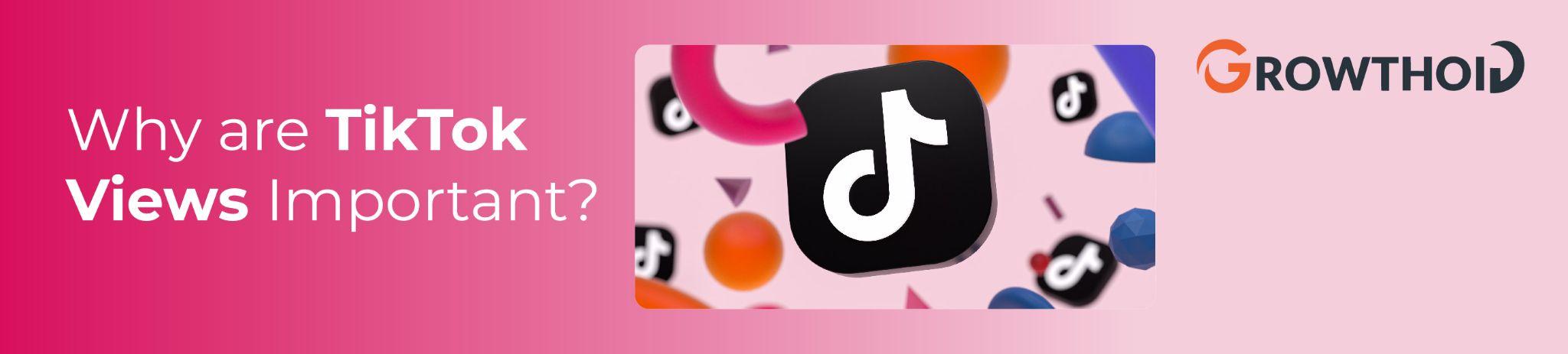The image is a horizontally oriented rectangle, approximately five times wider than it is tall. The background transitions from a deep, dark pink on the left, gradually lightening to a medium pink by the center, and continuing to a very light pink near the right, culminating in an almost white shade at the far right edge. 

Positioned about an inch down from the top and an inch over from the left edge, the text "YR" is displayed in white. Below it, in bolded white, the text reads "TikTok" on one line, followed by "Views" and "Important?" on the next line.

In the center of the image, there is another rectangle with a light pink background. This smaller rectangle contains four TikTok logo squares arranged with two on the left and two on the right. In the center of this grouping is a larger black square with the white TikTok 'T' logo.

Additionally, scattered within this central area are a few orange circles, some triangles, and several blue circles, adding visual interest.

To the right of this central rectangle, at the top, there is a stylized 'G' in green or orange. Beside this, "ROWTHOID" is written in bold, all capital black letters. Notably, the letter 'D' is uniquely designed, starting from the backside in a half shape that extends downward, loops up and around, and points off at the top left corner.